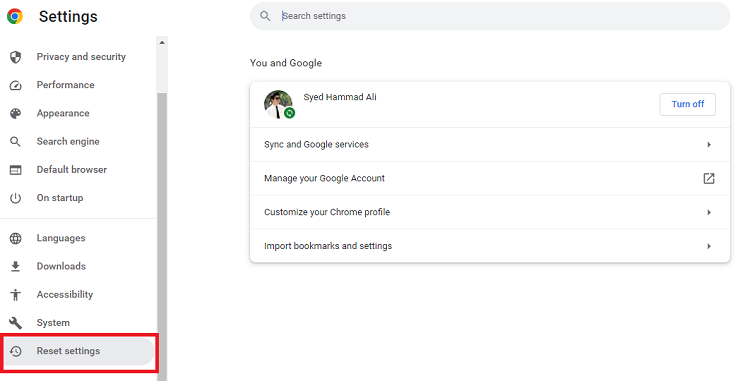This is a detailed screenshot of the Google Chrome settings page. On the left side of the screen, a toolbar labeled "Settings" is displayed alongside the Chrome logo—comprising the colors red, yellow, and green with a blue dot in the center, forming a circular shape. Below the toolbar, there are various categories listed: "Privacy and Security," "Performance," "Search Engine," "Default Browser," "On Startup," "Languages," "Downloads," "Accessibility," "System," and lastly "Reset Settings," which is grayed out and highlighted with a red box, indicating it is the currently selected section.

In the main content area of the page, there is a search bar at the very top labeled "Search settings" accompanied by a magnifying glass icon. Below this, a section titled "You and Google" is visible. It contains a user module featuring a profile picture and the name "Siad Hamed Ali." Next to the user profile is a green circular icon with two arrows, signifying active syncing. There is also an option to turn off this syncing feature.

Further down, there are various options including "Sync and Google services," "Manage your Google Account," "Customize your Chrome profile," and "Import bookmarks and settings." The remainder of the page is notably plain white, free of any additional text or graphics.